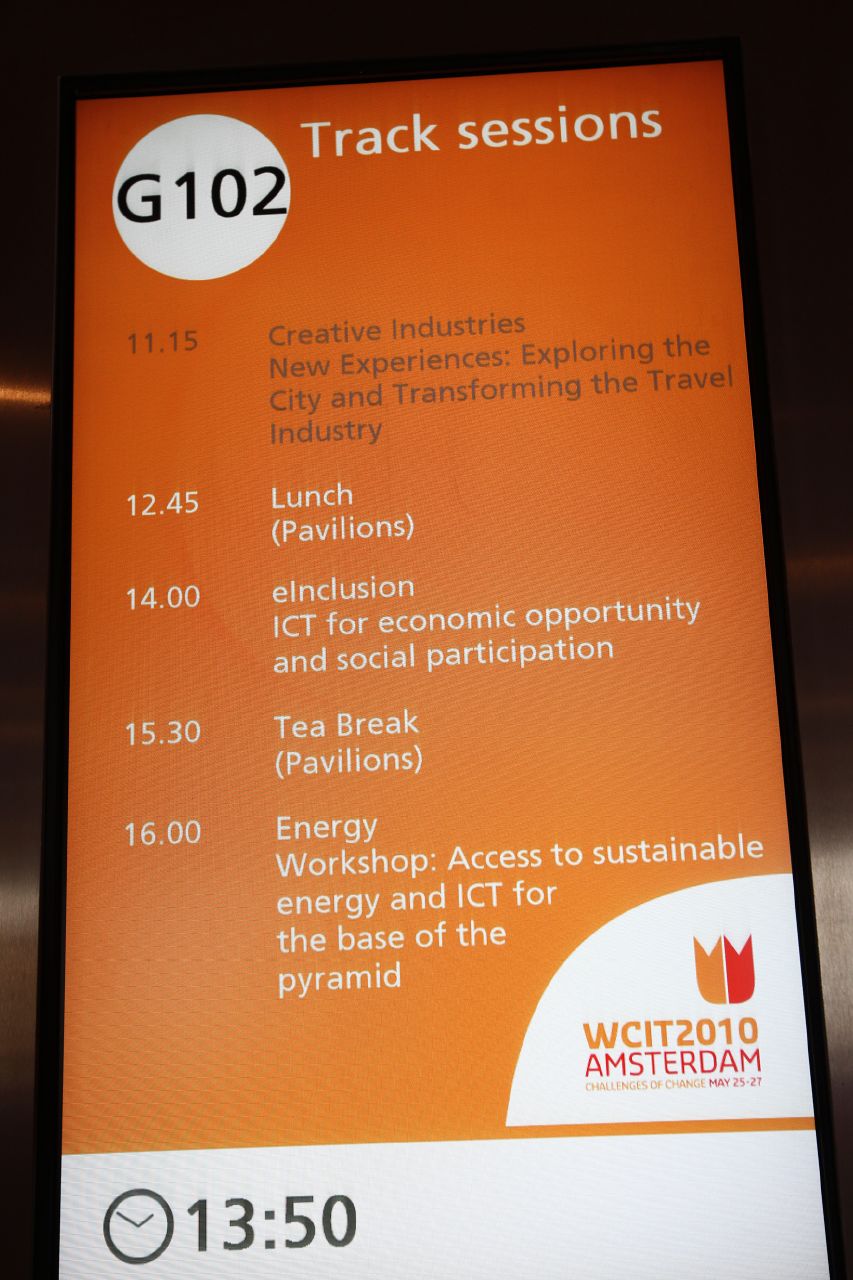The image features an orange and white digital sign, potentially mounted on a brown wall or placed atop a table. At the top left corner, a white circle contains the black text "G102." Next to it, in white text, it reads "Track Sessions." Below this heading, the sign lists a detailed schedule of events for a conference. The schedule begins with "11:15 - Creative Industries, New Experiences: Exploring the City and Transforming the Travel Industry” in gray text, followed by “12:45 - Lunch (Pavilions)” in white text. Continuing down, at “14:00 - E-Inclusion: ICT for Economic Opportunity and Social Participation,” followed by “15:30 - Tea Break (Pavilions),” and “16:00 - Energy Workshop: Access to Sustainable Energy and ICT for the Base of the Pyramid.” A clock icon at the bottom displays the time "13:50," and to the right, another circle indicates "WCIT 2010 Amsterdam," specifying the timing as May 25th through the 27th.